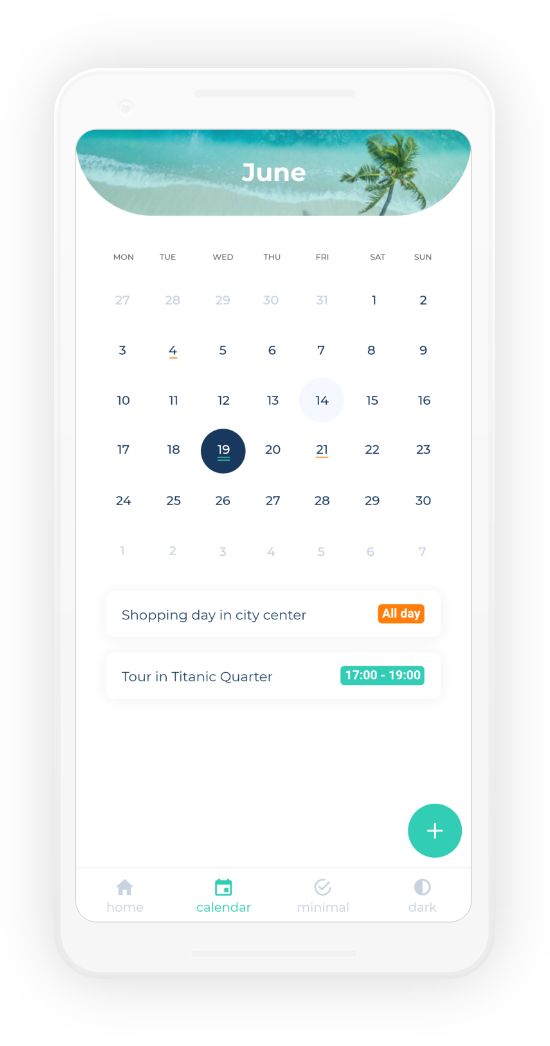A close-up shot of a calendar displays the month of June against a picturesque beach backdrop. The scene features a serene ocean with blue waters and a tall, lush palm tree. The calendar is organized with days of the week listed as Monday, Tuesday, Wednesday, Thursday, Friday, Saturday, and Sunday. The date range displayed includes the previous month's end (27 through 31), the current month of June (1 through 30), and the beginning of the next month (1 through 7) at the bottom. Noteworthy events are highlighted: "Shopping day in city center" spans all day, while "Tour in Titanic Quarter" is scheduled from 17:00 to 19:00. The calendar design includes a distinct white plus sign inside a green circle and a minimally darkened border at the bottom. Some dates and events are accentuated with a green background to emphasize their importance.